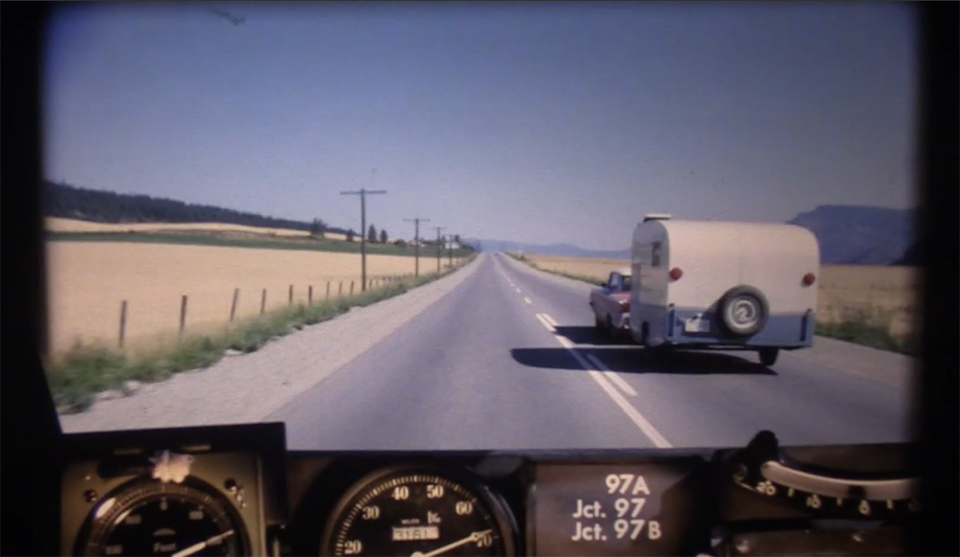This vintage photograph, likely from the 1970s or 1980s, captures a unique perspective from inside a vehicle, revealing the dashboard with a speedometer showing nearly 70 miles per hour and an odometer reading of 3161. The photo is taken from the driver’s seat, showcasing a red car on the right pulling a white and gray camper trailer down a rural highway. The road is flanked by green landscapes, with wooded areas and farm fields on the left, and rolling hills and mountains in the distance. Yellow planes are also visible, one on each side of the road, behind a fence on the left. The clear blue sky contrasts with the scenery, making the entire scene feel vast and open. The bottom right of the image displays numbers, including "97A," "Junction 97," and "Junction 97B," likely related to highway signage or navigation tools.